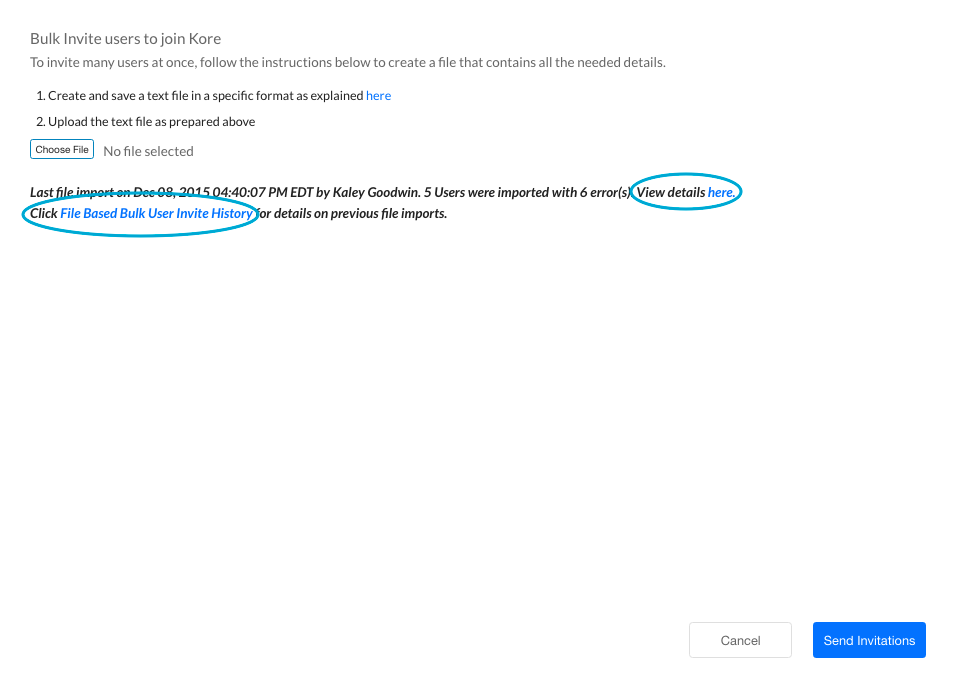The image showcases a message on a computer screen with a predominantly white background. At the top of the message, the header reads, "Bulk invite users to join KORE." The name "KORE" is uniquely spelled out in capital letters as K-O-R-E. Below the header, there are instructions for inviting multiple users simultaneously, which involves creating a specific file. 

The instructions are divided into two distinct steps:
1. "Create and save a text file in a specific format as explained here," with "here" being a clickable blue hyperlink.
2. "Upload the text file as prepared above," featuring a "Choose File" button with the text "No file selected."

Beneath these instructions, there is a section detailing the history of the last file import. It states, "Last file import on December 8th, 2015 at 4:40:07 PM EDT by Kaylee Goodwin," noting that five users were imported with six errors. The text "View details here" is included, with "here" also highlighted as a clickable blue link. This phrase is circled with a teal marker for emphasis.

At the bottom of the message, there is a link labeled "Click file based bulk user invite history," encircled with a teal marker, offering more details on previous file imports.